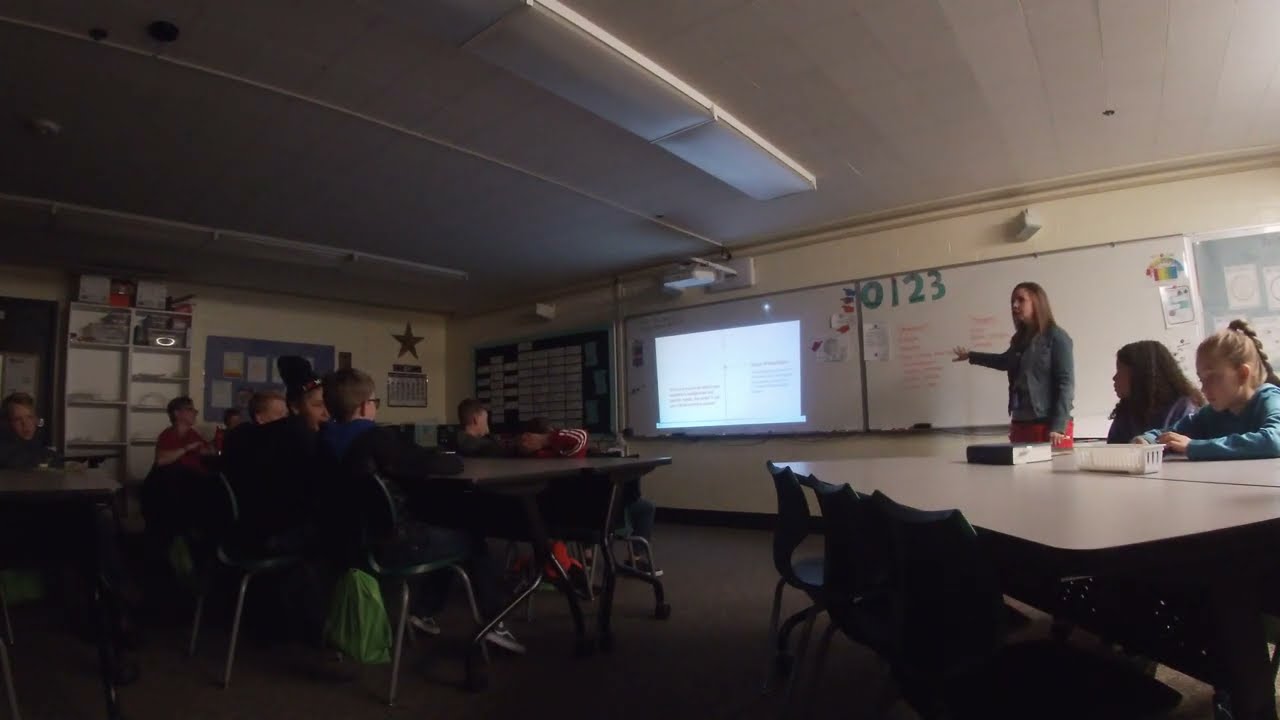The image depicts the inside of a children's classroom. The room is intentionally darkened to enhance the visibility of a projected image on a central whiteboard. The primary light source comes from the right side of the image. In the front, a teacher, dressed in a gray top and rose-colored pants or shorts, stands to the right of the projection with her arms outstretched, gesturing towards the displayed content. The whiteboard features green numbers "0, 1, 2, 3" with some red underlining. Most of the children are seated at communal tables or individual desks scattered around the classroom, engaged in working and attentively watching the projection. The classroom appears well-maintained, neat, and organized. To the right of the whiteboard, there is a blue bulletin board adorned with papers, and to the left, a wall at a 90-degree angle hosts a star decoration and possibly a shelving unit with utensils.